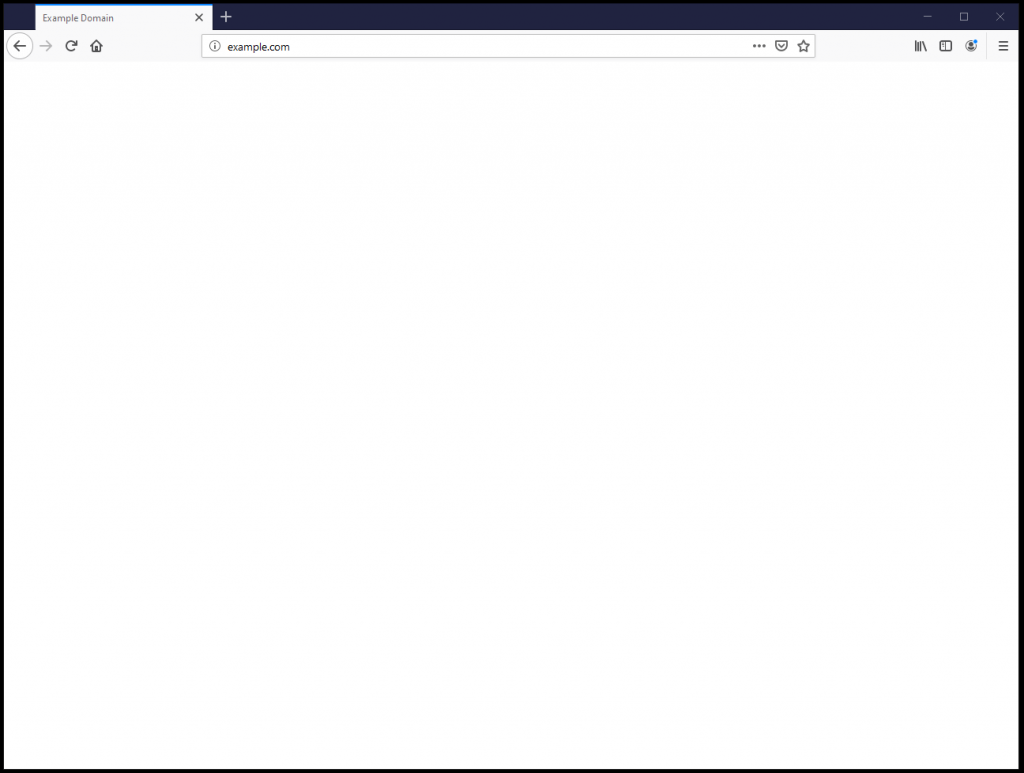The image depicts an empty web browser page. At the top left corner, the browser tab is labeled "Example Domain." Directly to the right of this, there is an "X" button, indicating the option to close the tab. Further along the row outside of the tab box, there's a "+" sign for adding a new tab. On the far right of the browser's top bar, there are three iconic buttons for window management: the "minimize" button, the "restore down" button, and the "close" button. Additionally, on the left side of the browser, there are navigation buttons with an arrow pointing left and another pointing right, followed by a "refresh" or "loading" button, and finally, a "home" button. The web page itself remains blank and devoid of content.